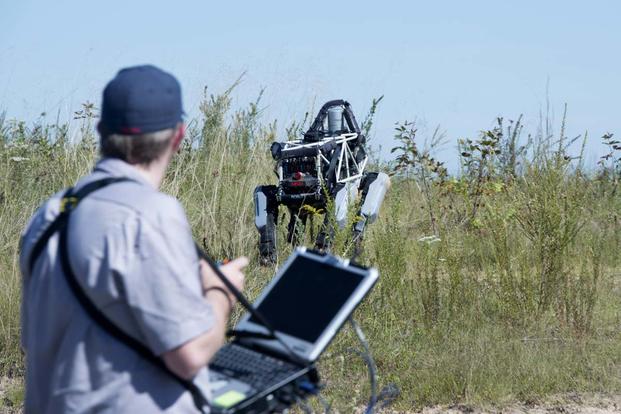In this outdoor image, a man in a blue collared shirt and a blue baseball cap stands in an overgrown, grassy field of wispy, beach-like weeds. The sky above is a clear, bright blue with some light clouds. The man has a laptop strapped to his front, its open screen and keyboard visible, suggesting he is using it to control or monitor a robot. The robot, a large, four-legged machine with a metallic build, features a roll cage on top with wires running along it, giving it a boxy appearance. The scene captures the man focused on the robot amidst the natural backdrop, with the robot poised in the tall grass.